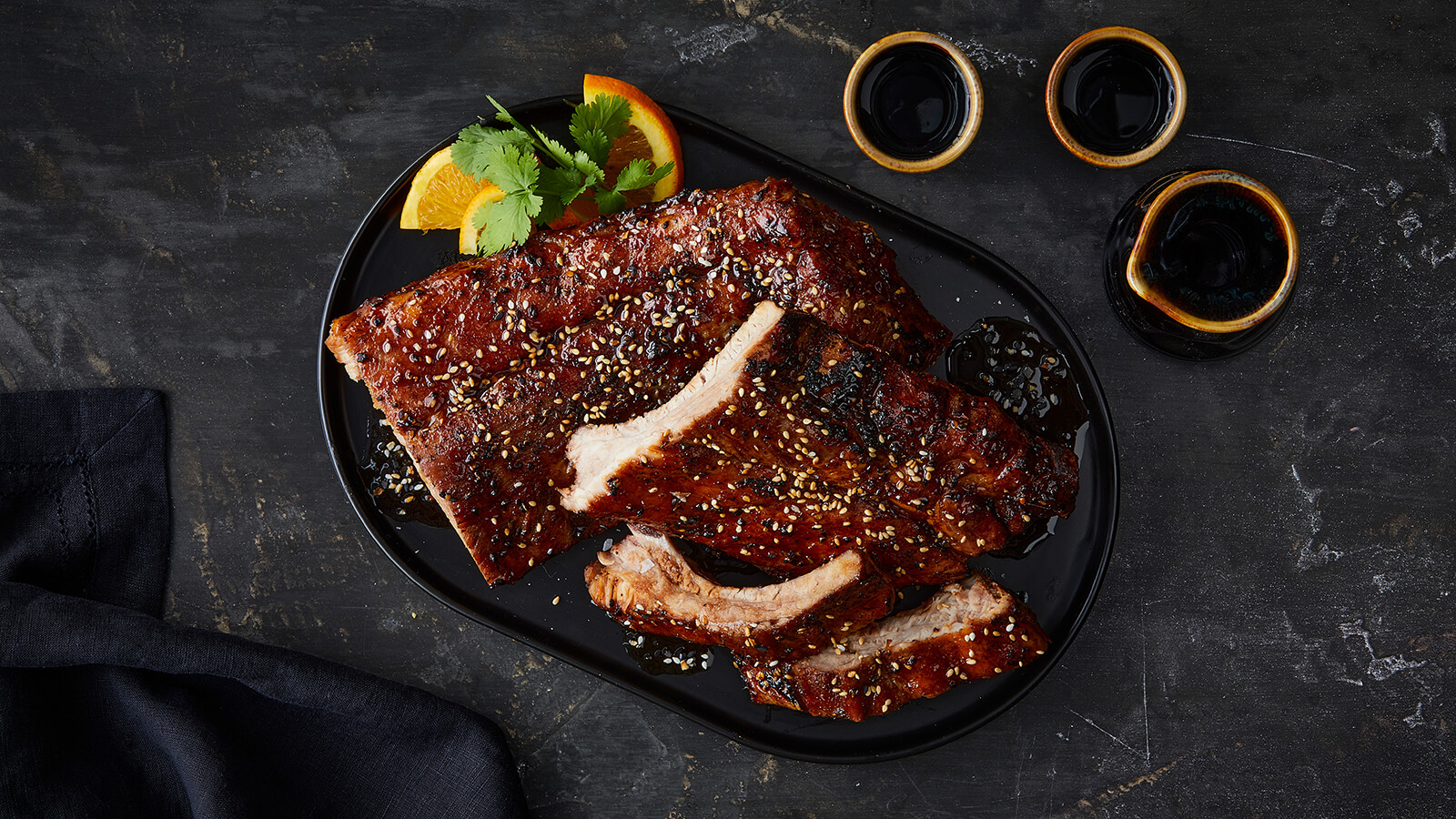This image is a detailed top-down view of a beautifully presented dish on a black oval plate with a subtle rim. The main focus is a rack of ribs cut in half, with two additional ribs separated from one half. The ribs are slathered in a rich, reddish barbecue sauce and sprinkled generously with sesame seeds. Garnishing the plate are vibrant slices of orange and sprigs of parsley, adding a refreshing touch of color to the savory presentation. The plate is positioned on a surface that resembles a chalkboard with flecks of tan, giving it a rustic yet sophisticated backdrop. In the bottom left corner, there’s a black satin napkin, adding to the elegance of the setting. Surrounding the main dish are three small black bowls with gold rims, each filled with a dark, delicious-looking barbecue sauce, complementing the succulent ribs perfectly.